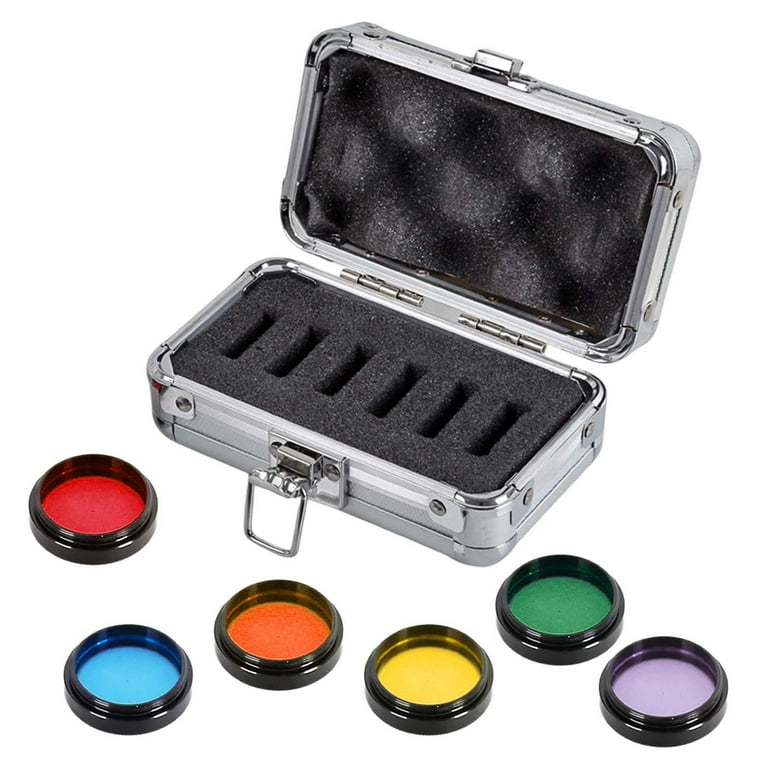The professionally photographed image features a sleek, open metal case with a silver exterior, set against a pristine white background. The interior of the case is lined with black foam padding, meticulously designed with six slots. Each slot cradles a small, black, circular disk filled with vibrant colors, likely intended for paint or makeup. From top to bottom and right to left, the colors displayed are red, light blue, orange, yellow, green, and light lavender purple. There is no text or branding visible in the image, accentuating the simplicity and focus on the colorful disks and the well-crafted case. This setup suggests the image is designed for promotional or advertising purposes.